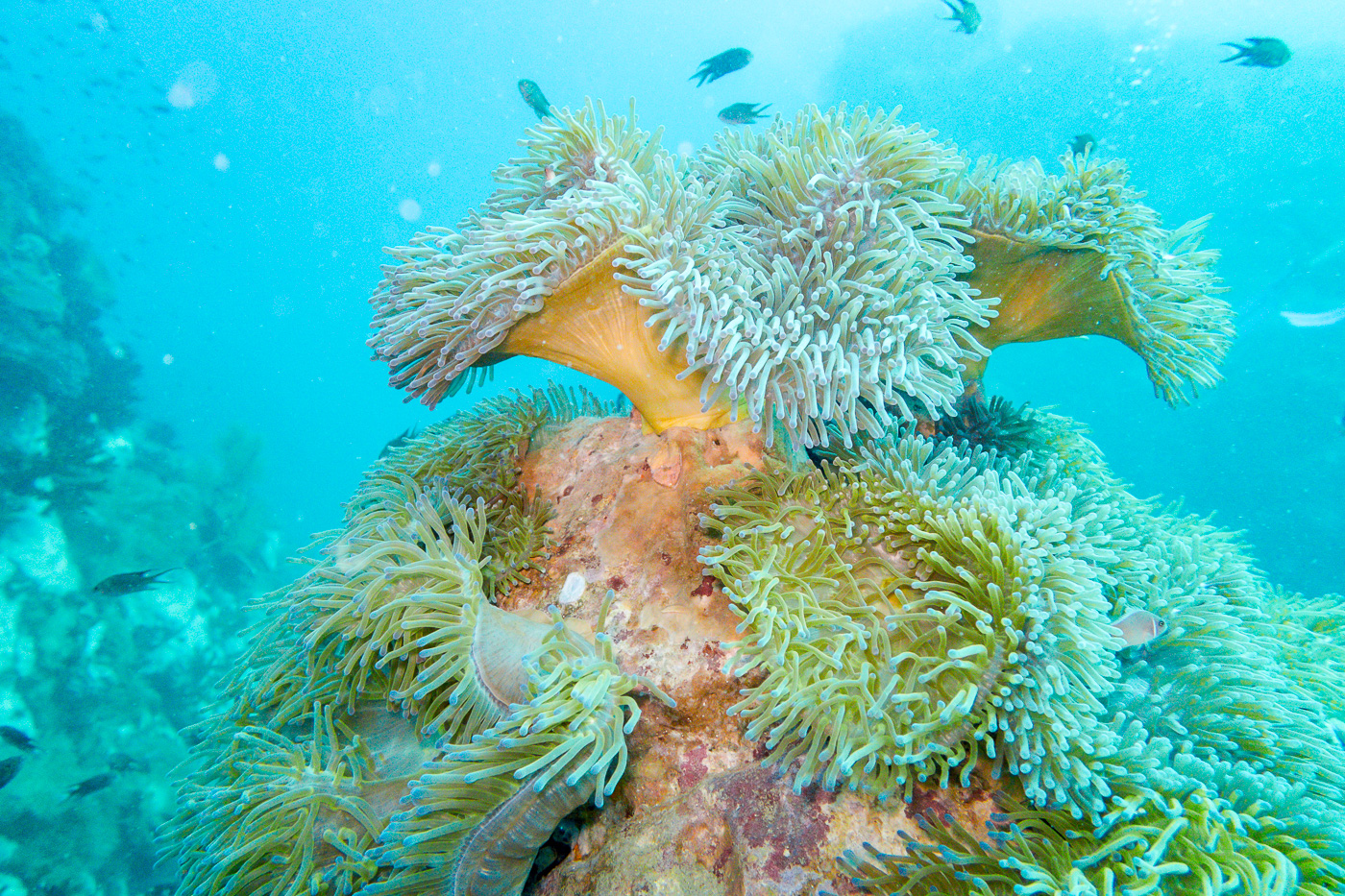The image showcases an underwater scene with a striking turquoise blue background. It features a horizontally oriented view of a coral reef teeming with life. Dominating the foreground is a large, peach-colored rock formation, adorned with fuzzy, spiny growths resembling anemone or sea urchins, giving it a lush, textured appearance. Dark-colored fish with long, pointed tails float lazily through the water, blending harmoniously with their vibrant surroundings. Smaller, lighter-colored fish can be seen swimming near the formations, while other rocks and underwater plants in the far background contribute to the rich tapestry of marine life. The entire scene is bathed in the serene hues of a turquoise ocean, offering a glimpse into the mesmerizing world beneath the waves.